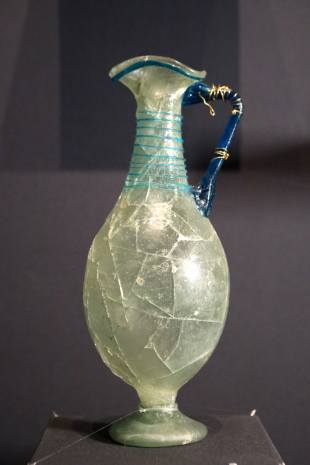This photograph captures an aged, semi-translucent vase, likely displayed in an art museum or gallery. The vase, made from a greenish jade-colored material, sits on a gray platform against a similarly gray background. It features a distinctive shape, narrowing at the neck, flaring at the top into a sort of spout, and expanding into a bulbous, pear-like bottom before tapering down to a small base. Cracks spiderweb across the vase's surface, adding to its historical charm. The handle, a striking deep blue, is adorned with gold wiring and contrasts sharply with the light blue, string-like material wrapped around its neck. This intricate wrapping continues in intervals down the neck, enhancing the vase’s elegant appearance.